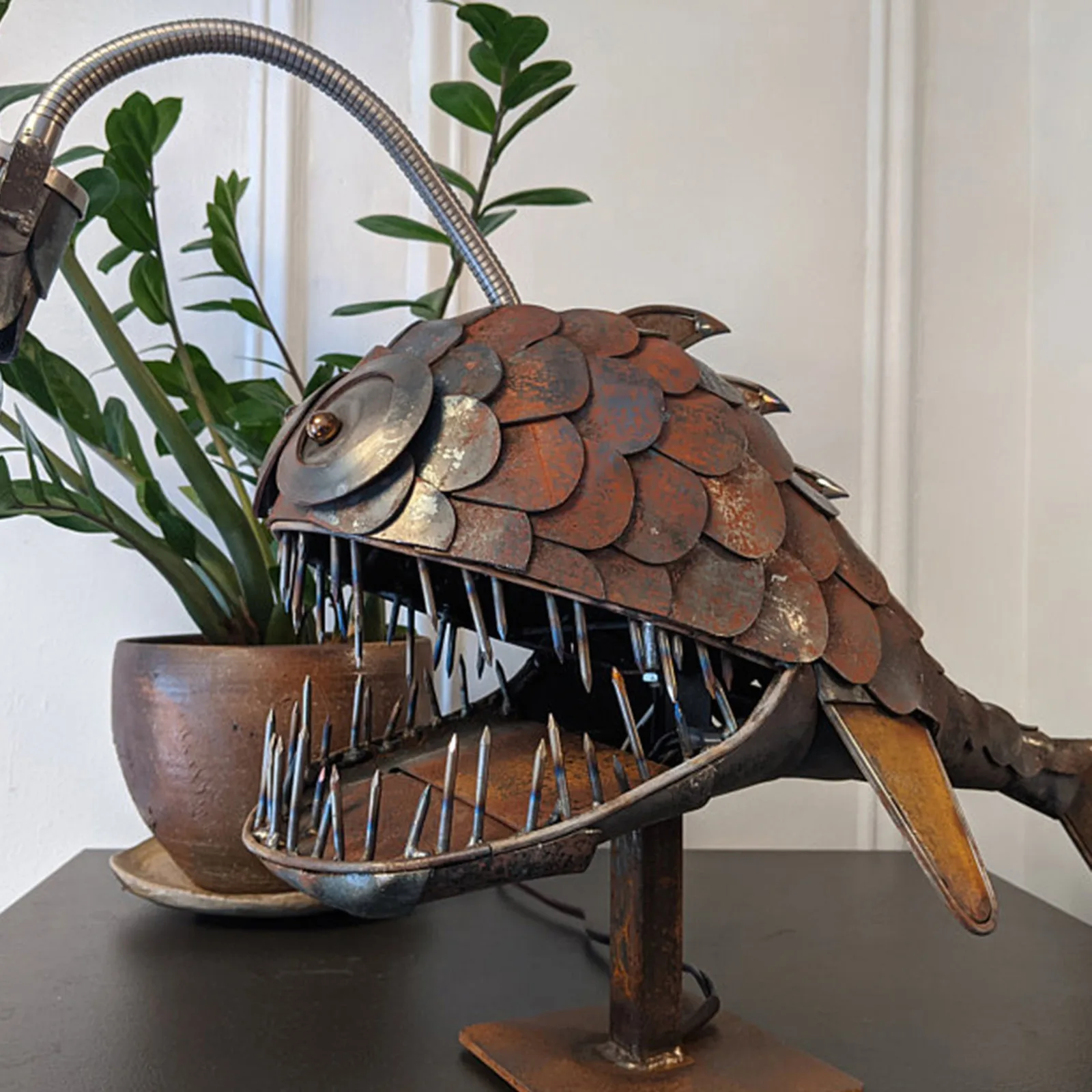The photograph shows a meticulously crafted welded metal sculpture of an anglerfish, set on a dark wood table against a white wall. The anglerfish features a very large head with an open mouth filled with sharp, pointy teeth, fashioned from nails. These nails have black lines, suggesting exposure to high temperatures. Overlapping round, rusty scales cover the top of the head, adding a touch of orangey-brown color. The sculpture boasts three spiky fins running down its back and a small fin protruding from the left side of its body. Prominently, there are two large circular eyes with 3D spherical pupils. A tall silver tube extends from the top of the head, resembling the lure of an anglerfish, likely ending in a light bulb, making the piece a lamp. The anglerfish is mounted on a vertical square pole that is welded into a square base. An extension cord runs through the center of the mouth and out of the base. In the background, a green potted plant adds a touch of nature to the scene.